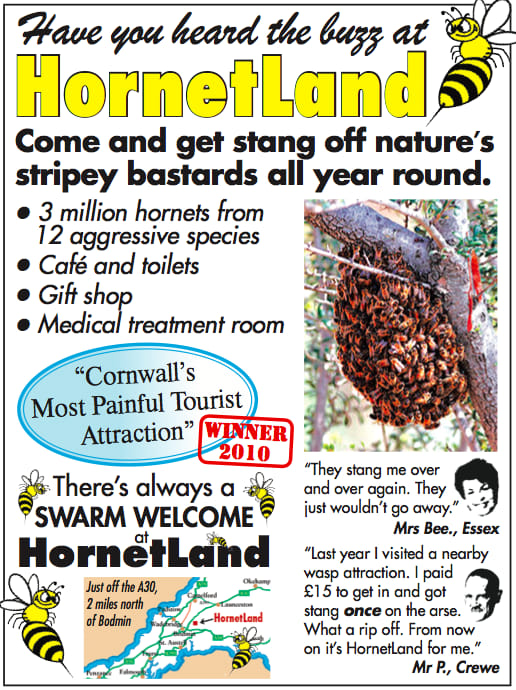This satirical poster advertises "Hornetland," Cornwall's most painful tourist attraction. The white background, bordered in black, features yellow letters for "Hornetland" and various cartoon hornets. The tagline, "Have you heard the buzz at Hornetland?" introduces the attraction where visitors can "get stung off nature's stripy bastards all year round." With three million hornets from 12 aggressive species, the site boasts a café, toilets, gift shop, and medical treatment room. A blue oval highlights the claim, "Cornwall's most painful tourist attraction," since Winter 2010. Located just off the A30, two miles north of Bodmin, the map and image of a hornet swarm on a tree branch underscore the experience. Visitor testimonials include Mrs. B from Essex, who said, "They stung me over and over again. They just wouldn't go away," and Mr. P from Crewe, who switched to Hornetland after a disappointing visit to a wasp attraction where he paid £15 and got "stung once on the arse."